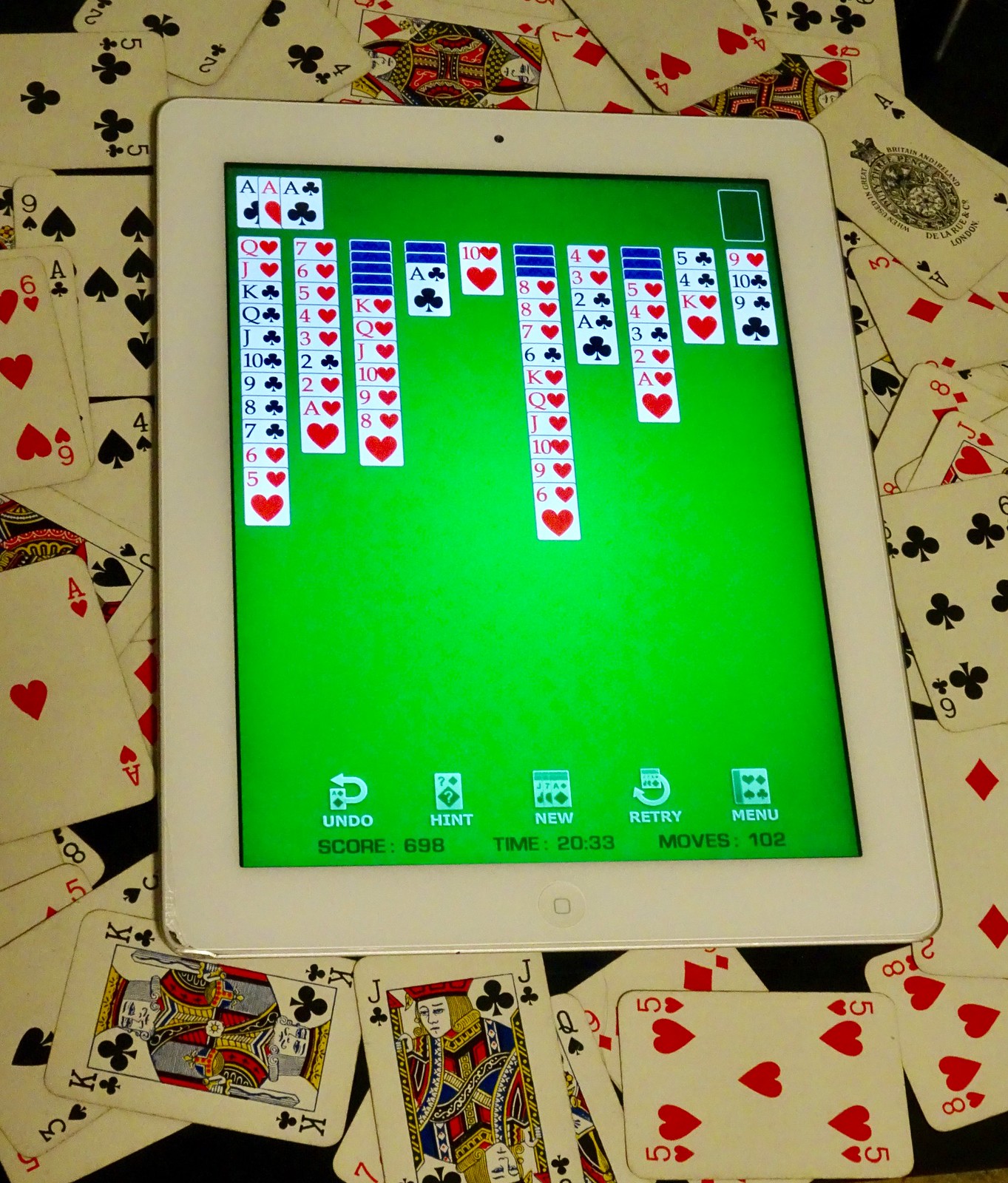The photograph features a computer tablet displaying an online card game. The game's interface is set against a green background, with several vertical columns showcasing spread-out cards. At the bottom of the screen, various icons are visible, including options for undo, hint, new game, retry, and menu. Below these icons are the game statistics: a score of 698, time elapsed at 20:33, and a total of 102 moves made. 

The tablet is placed on a surface nearly buried under a cluttered assortment of physical playing cards, featuring all suits—spades, hearts, diamonds, and clubs. The playing cards appear well-worn, with noticeably discolored edges, suggesting frequent use. The surface underneath these cards and the tablet is black, possibly a table or a bed covered in a dark fabric. The scene conveys a blend of digital and physical gaming, highlighting a rich tapestry of play and nostalgia.